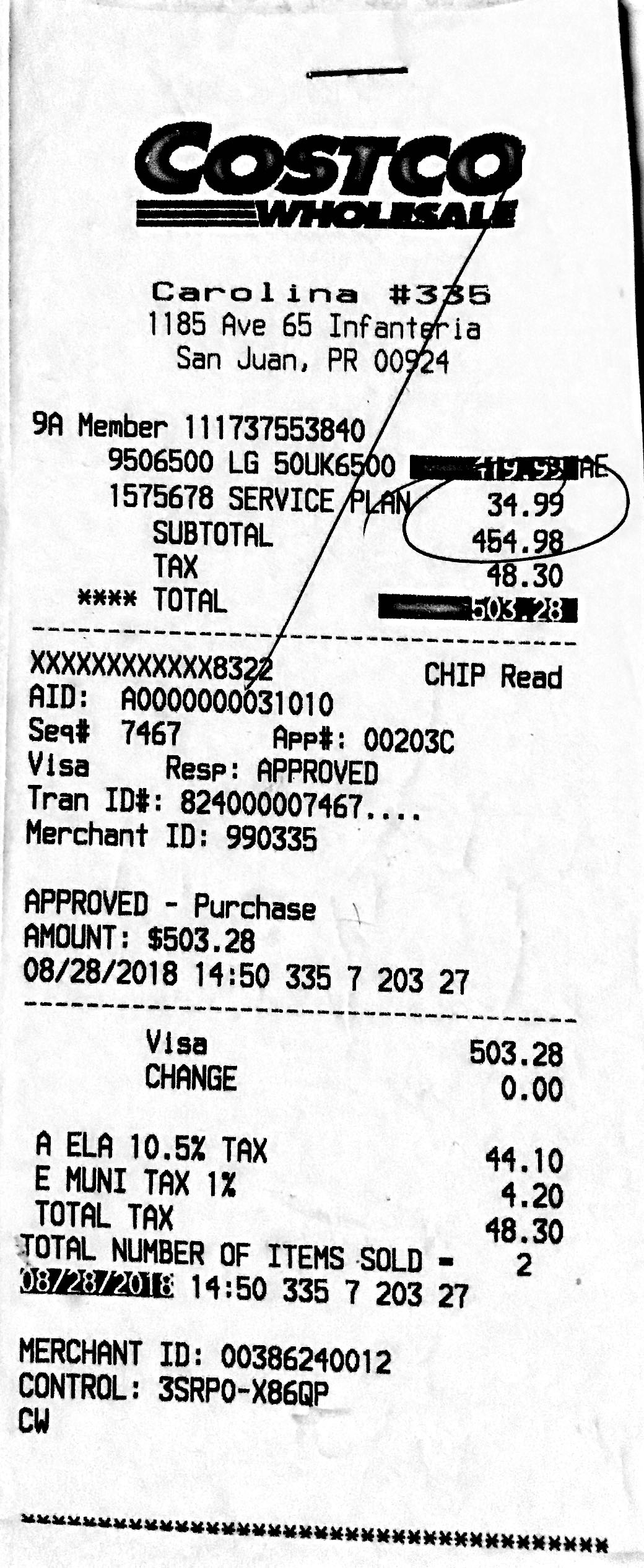This image is a detailed picture of a white sales receipt from a Costco Wholesale store, specifically from the Carolina location, store number 335, situated at 1185 Avenue, 65 Infanteria, San Juan, Puerto Rico, 00924. The store details are prominently printed at the top in bold black text. The receipt documents a purchase made on August 28, 2018, at 14:15, totaling $503.28, paid via Visa. The items listed include an LG sound system priced at $499.99 and a service plan costing $34.99. The subtotal for these items is $534.98, with additional taxes detailed as follows: $44.10 in local tax and $4.20 in Muni tax, summing up to a total tax of $48.30. The receipt further notes it was an approved chip read transaction. The membership number associated with the purchase is 111-737-553840.